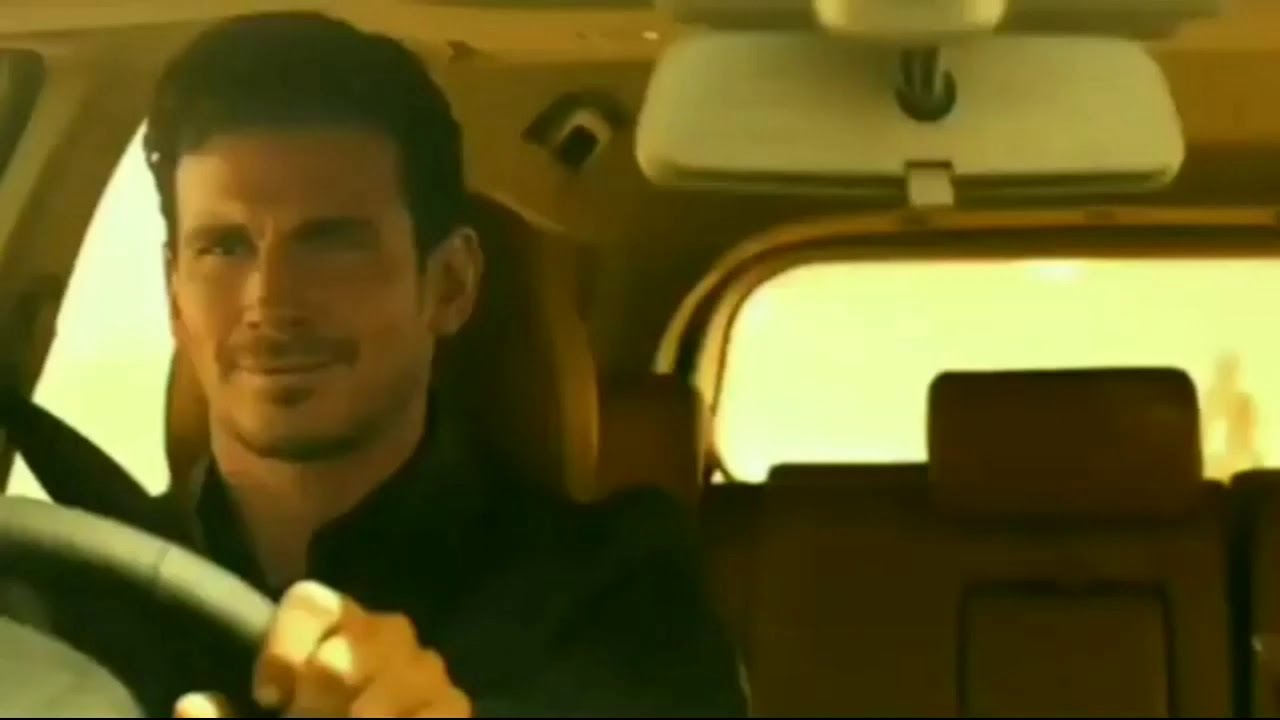This is a color photograph of a man driving a car, taken from the dashboard or through the windshield. The man, positioned on the left side of the image, has dark brown hair and light facial scruff, including a mustache and partial beard. His left hand grips the gray steering wheel, visible in the lower left corner, with a bit of his seat belt also in view. He is wearing a black collared shirt and appears to have a closed mouth with a subtle, perhaps sneaky-looking expression.

The rear view mirror, which is white in color, is visible in the upper right corner. The back seat and rear window occupy the right middle half and lower right quadrant of the image. The car features brown leather upholstery, noticeable in both the headrest and the back seat. There doesn't seem to be any other passengers visible in the vehicle. Outside the windows to the man’s left and visible in the rearview mirror, there are yellow hues with indistinct shadowy figures. The car's headliner is a light brown color. Overall, the image is slightly blurry and suggests it might be a sunny day.